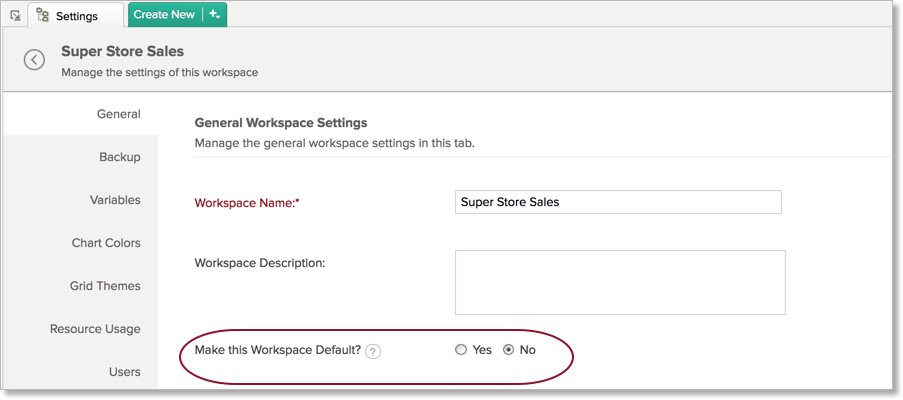The image displays a webpage with a rectangular, gray interface. At the top, there are two tabs labeled "Settings" and "Create New," with the latter tab highlighted in green. Beneath the tabs, the header "Superstore Sales" is prominently displayed, followed by the subheading "Manage the settings of this workspace." 

On the left side of the webpage, there is a vertical navigation menu. The menu includes the following options listed sequentially: "General" (highlighted), "Backup," "Variables," "Chart Colors," "Grid Themes," "Resource Usage," and "Users." Each option is aligned vertically, facilitating easy navigation.

To the right of the navigation menu, the text "General Workspace Settings" is displayed in bold. Below this, a description reads "Manage the general workspace settings in this tab." 

In the center of the page, there is an empty input box with red text marked by an asterisk, labeled "Superstore Sales." Below this input box, another field titled "Workspace Description:" is present, followed by a second empty box for input.

Near the bottom of the image, the phrase "Make this workspace default?" is shown with an accompanying question mark icon. Following this, there are clickable 'Yes' and 'No' bubbles designed for selection, with the 'No' bubble currently selected. This section is prominently outlined by a red oval, drawing attention to it.